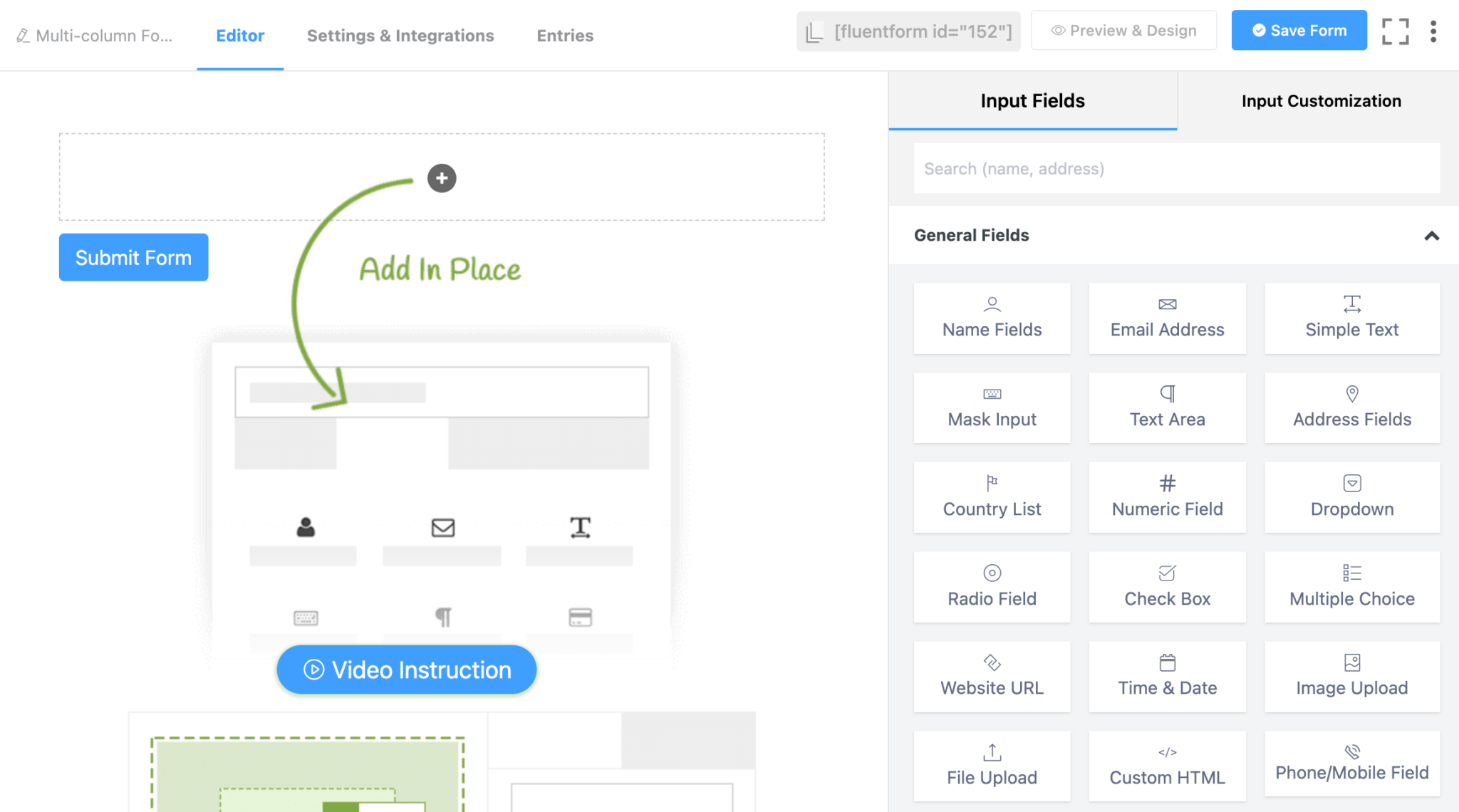The image displays a software interface for a multi-column editor with various settings and integration options. At the top, "Multi-Column Editor" is prominently highlighted in blue. To the right, the menu includes options such as "Settings and Integrations," "Entries," "Preview and Design" (highlighted in grey), and "Save Form" (highlighted in blue). Adjacent to these, there's a square icon containing three dots and a plus sign within a box labeled "Add in Place" in green. To the left of the plus sign, there's a "Submit Form" option. Below the plus sign, there is an area where you can add elements, featuring a blue circle that includes the text "Video Instructions" and a play button. 

A green box with dotted lines is partially cut off, making its text unidentifiable. Adjacent to this, the interface lists "Input Fields" and "Input Customization" in black text, accompanied by a search bar labeled "Name or Address." Available input options include:

- Name Field
- Mask Input
- Country List
- Radio Button
- Web URL
- File Upload
- Email Address
- Text Area
- Numeric Field
- Checkbox
- Time and Date
- Custom HTML
- Simple Test
- Address Field
- Drop-down
- Multiple Choice
- Image Upload
- Photo
- Mobile Field